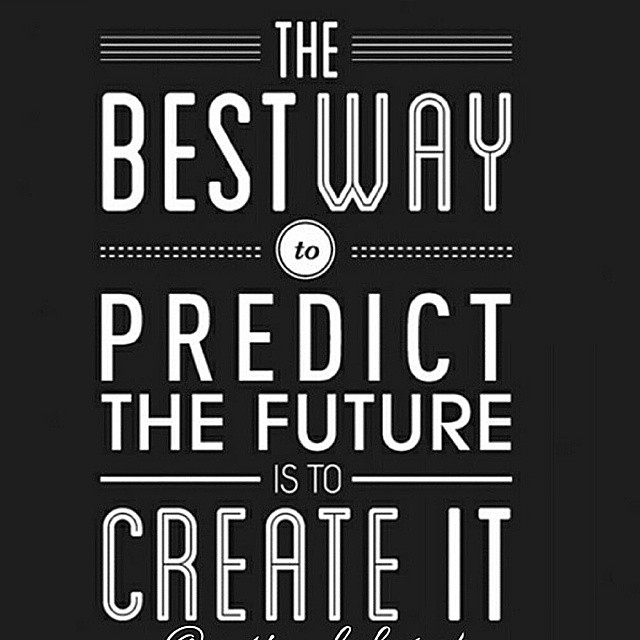This image features an inspirational quote in a square format with a slightly taller height than width. The background is solid black, emphasizing the white text that reads: "THE BEST WAY TO PREDICT THE FUTURE IS TO CREATE IT." The text is arranged with each word in a different font, creating an artistic and visually engaging presentation. At the top, "THE" is in uppercase letters, followed by "BEST WAY" in larger font. The word "TO" appears in small black letters inside a white circle, surrounded by dotted lines. Below this, "PREDICT" stands out in big letters, followed by "THE FUTURE" in slightly smaller font. The phrase concludes with "IS TO CREATE IT" in a mix of larger and smaller letters, maintaining the stylistic theme. Horizontal and dotted lines are thoughtfully placed around the text, adding to the balanced, artistic feel of the entire composition.